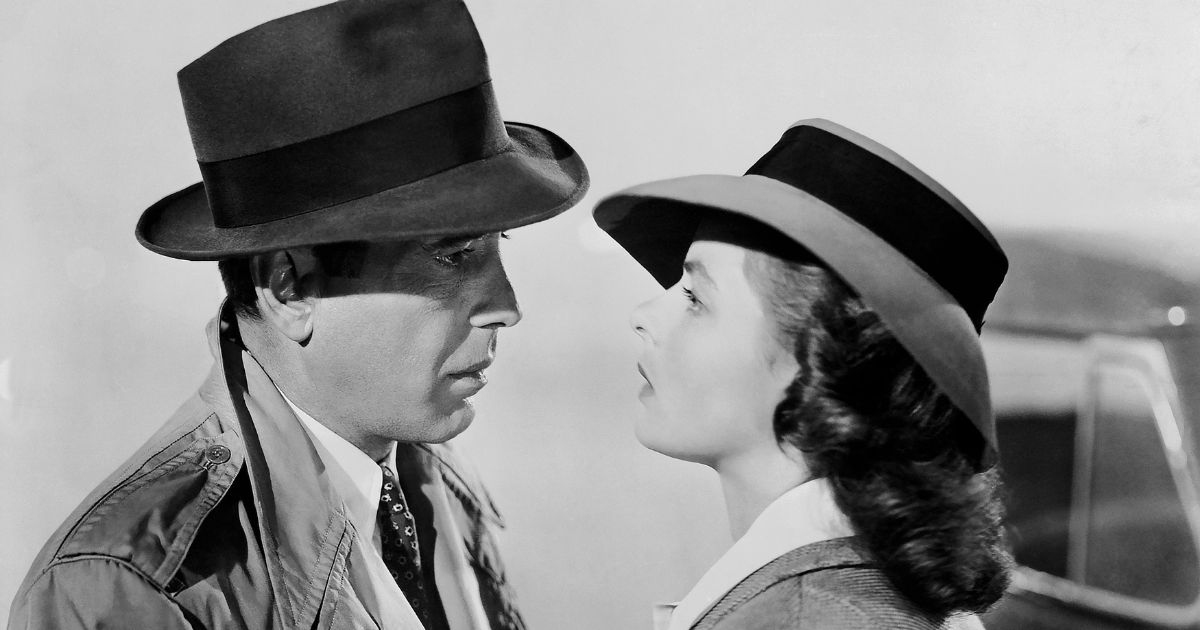In this black-and-white photograph, which appears to be a still taken from the end of the movie "Casablanca," we see Humphrey Bogart and Audrey Hepburn standing close together, exuding deep affection. The predominantly grayscale image captures a moment of intimacy as their hat brims nearly touch. Bogart, positioned on the left, wears a dark, black hat with a black stripe, a long trench coat, a white dress shirt, and a necktie adorned with circular patterns. His dark hair peeks out slightly from under his hat. Hepburn, on the right, dons a grey hat with a black stripe, her dark, shoulder-length hair curled at the ends. She is in a jacket with a white collar, looking intently at Bogart. In the background, to the right of Hepburn, the outline of a car window and car top adds depth to the scene. Both characters seem immersed in a passionate gaze, conveying a palpable sense of love and connection.